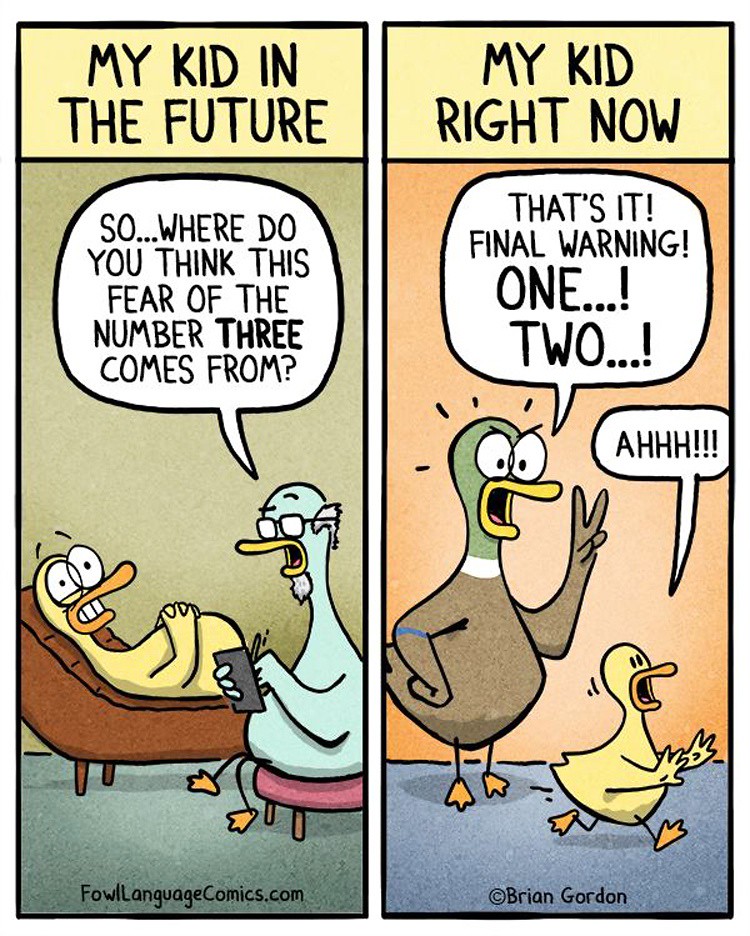The image is a two-panel comic strip with a yellow rectangular box at the top of each panel. The left panel is captioned "My Kid in the Future" in black text. It features an old duck sitting on a chair, interviewing another duck that is reclining. The speech bubble above the old duck reads, "So, where do you think the sphere of the number three comes from?" At the bottom left, there's a website link, "FOWLLANGUAGECOMICS.COM". The right panel, captioned "My Kid Right Now," shows a brown duck yelling at a kid duck with two speech bubbles saying, "That's it, final warning, one, two." The kid duck, depicted as a yellow duck, is running away while exclaiming, "Ahhh!" The comic is created by Brian Gordon. The background of both panels is predominantly gray, accentuating the yellow of the rectangular captions at the top. The characters are all anthropomorphic ducks, with distinct colors and expressions illustrating the humorous contrast between the imagined future and the present reality of parenting.